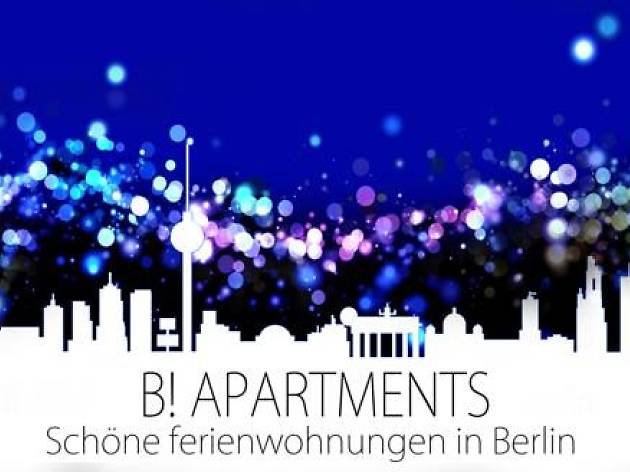The image is a vibrant advertisement for B! Apartments in Berlin. It features a bold graphic design with a dominant blue background filled with floating bubbles in shades of blue, purple, pink, and white. The lower section of the image depicts a white silhouette of Berlin's skyline, showcasing various buildings including skyscrapers, some topped with antennas, domes, and columns. At the bottom of the image, in black text against the white backdrop, the words "B! APARTMENTS" stand out prominently in uppercase letters. Below this, a German phrase "Schoneferienwohnungen in Berlin," translates to beautiful holiday apartments in Berlin, emphasizing the city's offerings. The dynamic artwork and detailed urban skyline create a striking visual promoting apartment living in Berlin.